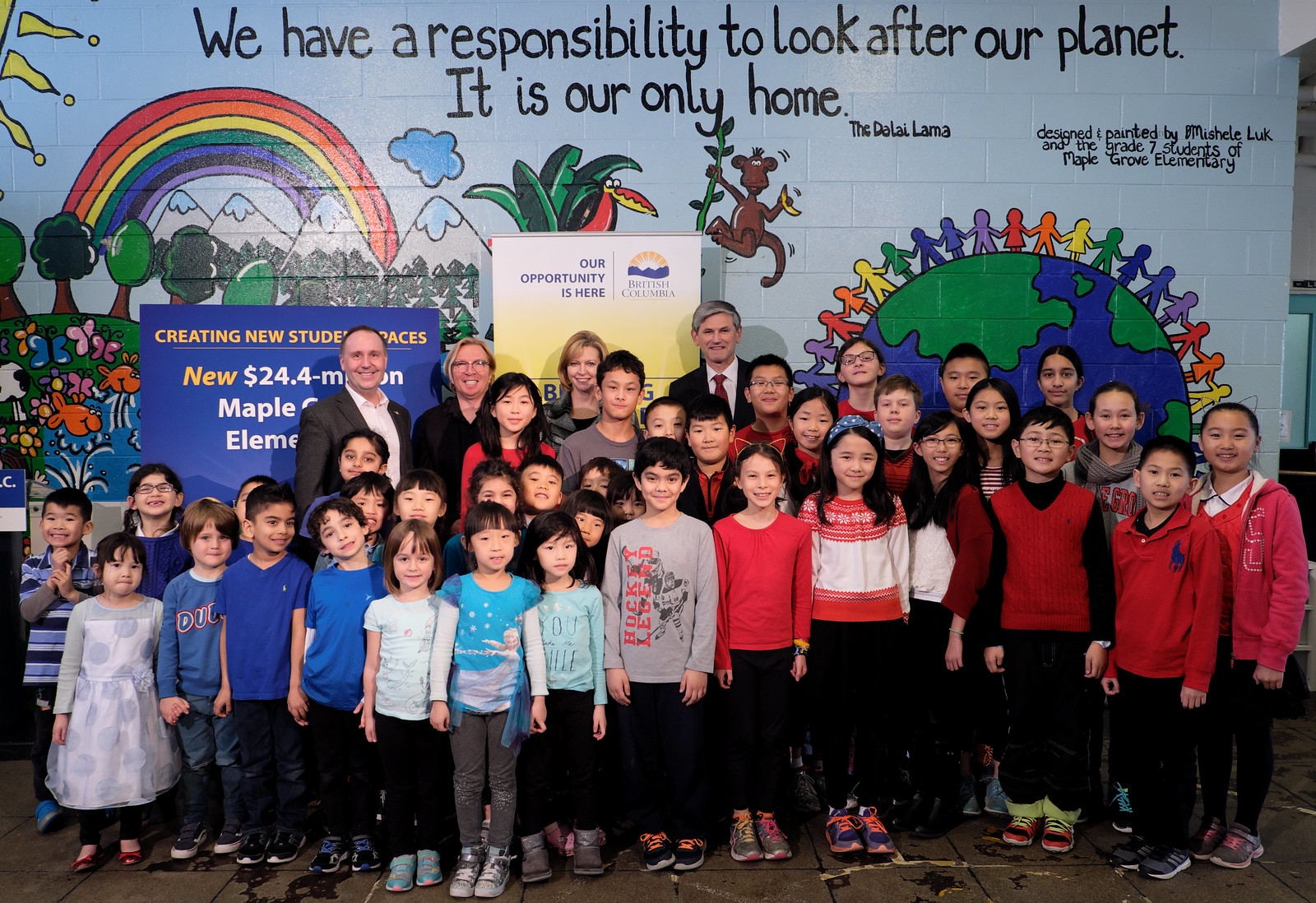In the image, a group of approximately 20 young children, primarily of Asian descent and around six or seven years old, are posed for what appears to be a class or group picture. They are dressed casually while standing in front of a vibrant mural painted on a light blue brick wall. The mural features various elements, including a central depiction of the Earth encircled by multicolored people holding hands, symbolizing unity. To the left of this, a rainbow arcs over mountains and trees, and a sun is visible in the upper left corner. In the center of the mural, a monkey holding a banana is perched on a branch above a pelican standing in some grass. The mural bears the inscription, "We have a responsibility to look after our planet. It's our only home," attributed to the Dalai Lama. Additionally, on the right side of the mural, a dedication reads, "Designed, painted by Michele Luke and the 7th grade students of Mabel Grove Elementary." Four middle-aged adults, dressed in professional business attire, stand behind the group of children, enhancing the formal atmosphere of the scene.